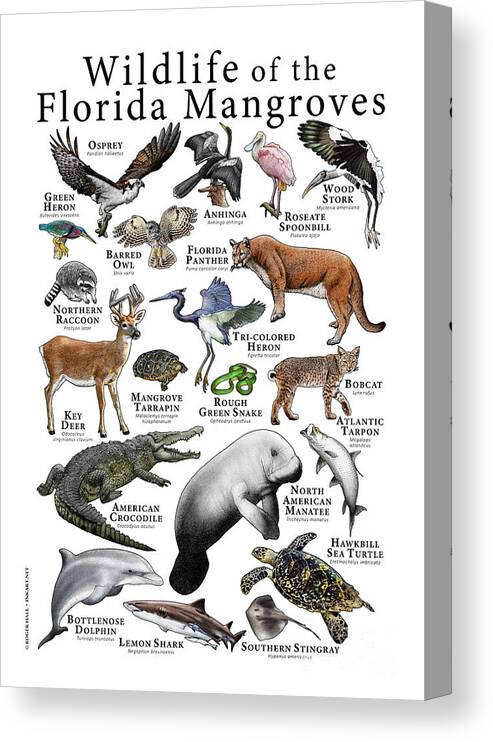The image is a detailed, three-dimensional poster titled "Wildlife of the Florida Mangroves," set against a white background with grey edges adding depth, resembling an artwork mounted on a canvas. The top of the poster prominently features the title in black font. Below, various Florida mangrove wildlife illustrations are meticulously labeled with their names, showcasing a wide variety of species. These include both terrestrial and aquatic creatures: the osprey, anhinga, roseate spoonbill, wood stork, green heron, barred owl, Florida panther, northern raccoon, key deer, mangrove terrapin, rough green snake, tricolored heron, bobcat, Atlantic tarpon, American crocodile, North American manatee, bottlenose dolphin, lemon shark, southern stingray, and hawksbill sea turtle. Each animal is depicted in its natural colors, adding to the visual appeal and educational value of the poster, highlighting the biodiversity of Florida's mangrove ecosystems.